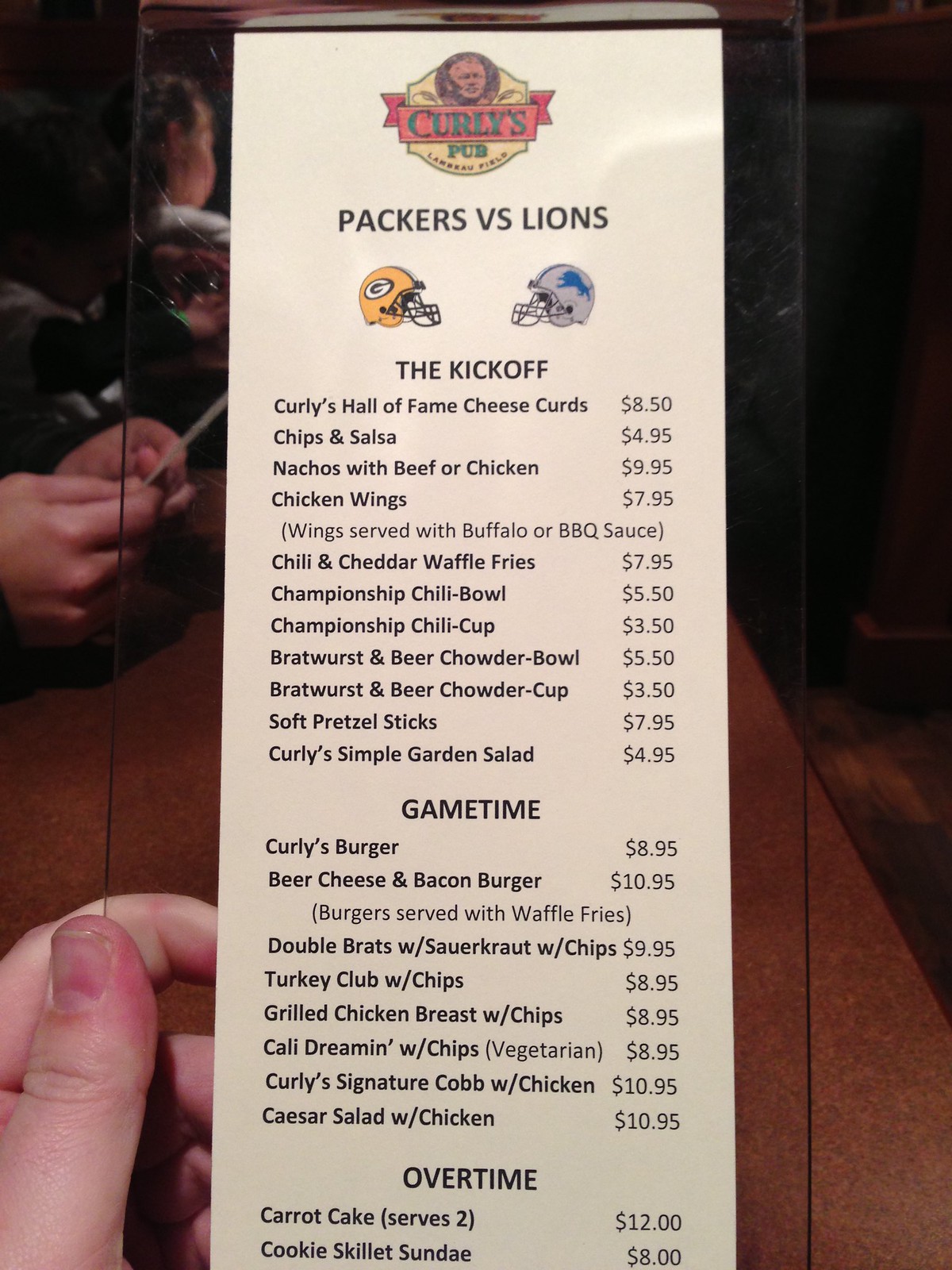The photograph captures a moment at Curly's Pub, where a person of Caucasian descent is holding a tall, rectangular glass menu in the foreground, positioned in the bottom left corner so that their thumb and the undersides of their fingers are visible. The menu, encased in glass, features an off-white or beige paper inside. At the top of the menu, "Curly's Pub" is prominently printed, accompanied by an illustration of the Egyptian pyramids in brown. Below this header, the text "Packers vs. Lions" is displayed, flanked by the helmets of the Green Bay Packers on the left and the Detroit Lions on the right. The Packers helmet is yellow, while the Lions helmet is gray with a blue lion logo. Beneath this section, the word "Kickoff" is centered, guiding diners to a list of available foods and their prices. 

The menu is divided into sections: 

- **Curly's Hall of Fame**: Cheese Curds $8.50, Chips and Salsa $4.95, Nachos with Beef or Chicken $9.95, Chicken Wings (with Buffalo or Barbecue Sauce) $7.95, Chili and Cheddar Waffle Fries $7.95, Championship Chili Bowl $5.50, Championship Chili Cup $3.50, Bratwurst and Beer Chowder Bowl $5.50, Bratwurst and Beer Chowder Cup $3.50, Soft Pretzel Sticks $7.95, Curly's Simple Garden Salad $4.95
- **Game Time**: Curly's Burger $8.95, Beer Cheese and Bacon Burger (served with Waffle Fries) $10.95, Double Brats with Sauerkraut and Chips $9.95, Turkey Club with Chips $8.95, Grilled Chicken Breast with Chips $8.95, Cali Dreamin' (Vegetarian, served with Chips) $8.95, Curly's Signature Cob with Chicken $10.95, Caesar Salad with Chicken $10.95
- **Overtime**: Carrot Cake $2.00, Cookie Skillet Sundae $8.00

Some of the prices and item names may vary slightly due to different interpretations in the captions, but this detailed description encapsulates the essence of the visual and textual information provided across all three descriptions.